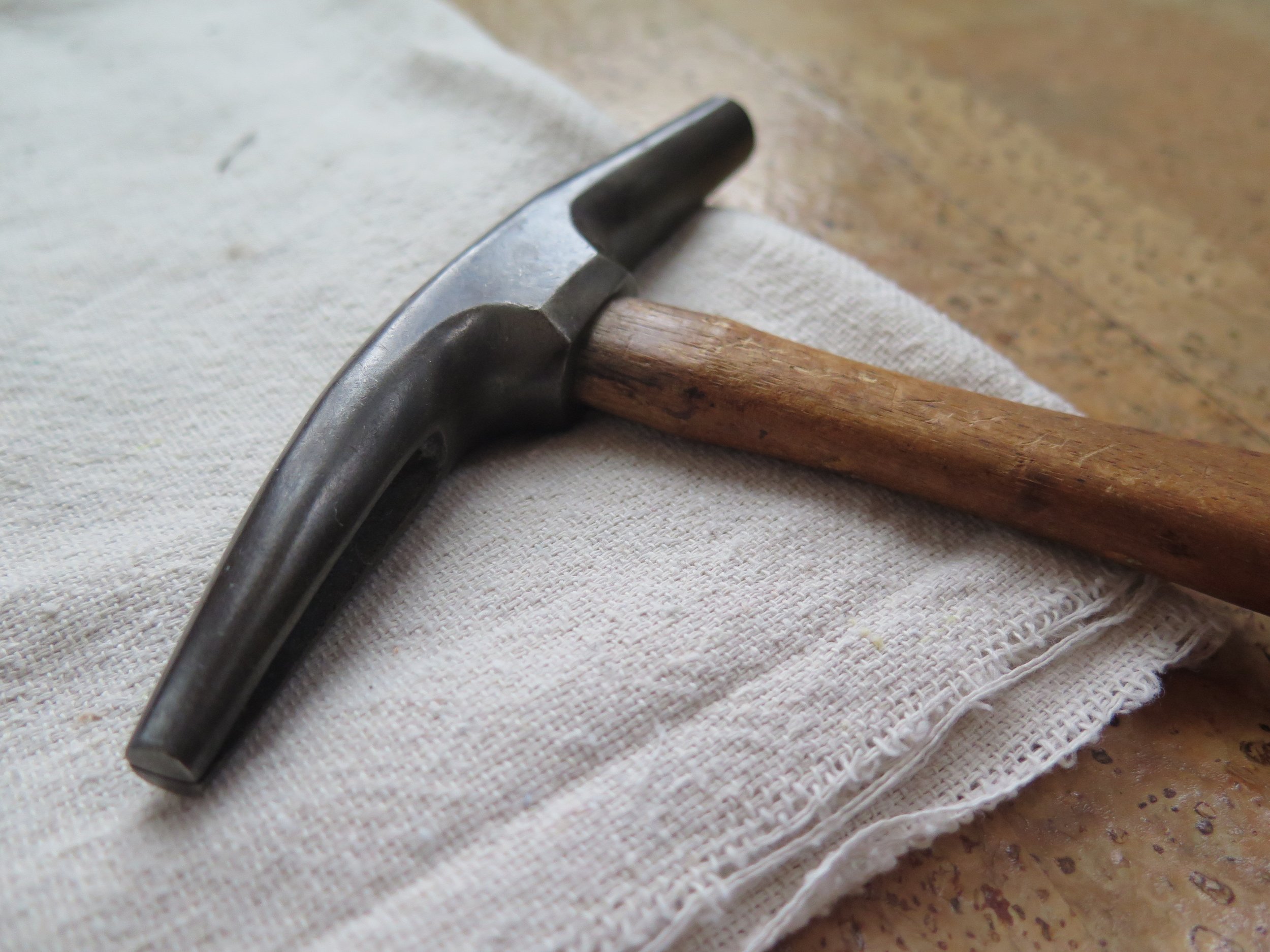The photograph captures a close-up of a folded, loosely woven white cloth placed on a tan travertine surface, possibly a countertop or floor. Resting atop the cloth is a distinctive tool, initially puzzling in its identity. The device resembles a walking cane handle at first glance, but closer inspection reveals it to be a uniquely shaped rock hammer. The hammer features a wooden handle that is slightly darker than the travertine background, extending into a sturdy steel head. The metal head is designed without claws and has a long, tapering design ideal for precise rock tapping, reminiscent of a geologist’s or hobbyist’s tool. The intricacies of the cloth, stone surface, and specialized tool combine to create an image rich in texture and subtle detail.